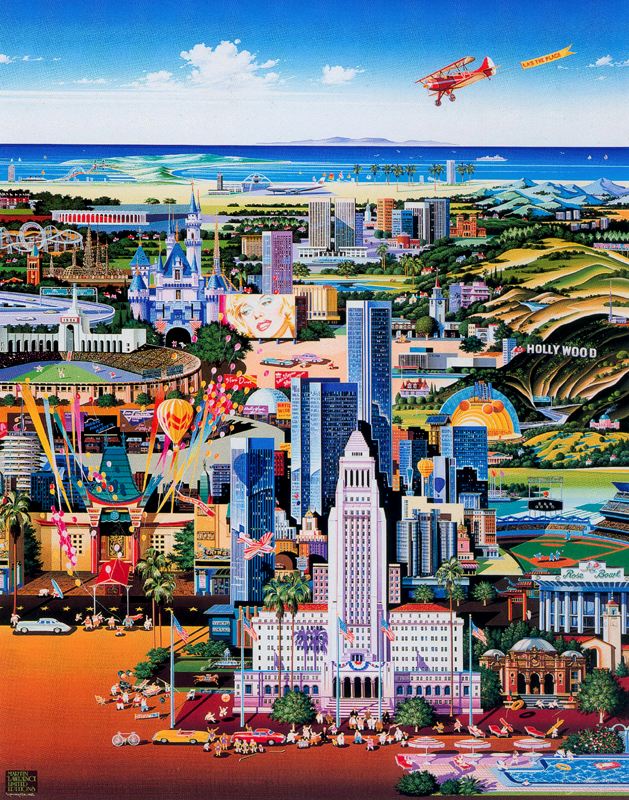This vivid artwork presents a bustling, dream-like cityscape filled with a kaleidoscope of bright, vibrant colors. Dominated by towering skyscrapers and various buildings both big and small, the image is a rich collage of diverse elements. In the foreground, there is a swimming pool positioned in the bottom right, adding a touch of leisure. Skyscrapers in white and blue, likely depicting glass buildings, rise prominently in the center. 

To the left, a stadium, which could be either a baseball or football field, is easily identifiable, while the iconic Hollywood sign decorates a hillside to the right. Amidst this colorful chaos, a hot air balloon floats, and a river meanders under an arch of trees. 

The middle section flaunts a giant TV screen displaying an image of Marilyn Monroe, or perhaps Debbie Harry, adding a touch of vintage Hollywood glamour. A red airplane, reminiscent of old-fashioned Wright Brothers models, soars through a partially cloudy, blue sky carrying an undecipherable banner. Surrounding this, a rollercoaster, churches, mosques, and a beach lined with palm trees populate the scene, along with bustling cars and pedestrians navigating the streets below.

Mountains and hills create a backdrop against the blue body of water stretching across the horizon. This colorful, busy rendition of California and Hollywood blends elements ranging from castles to different architectural styles, capturing the eclectic vibrancy of a city where everything seems just slightly out of scale, akin to a whimsical collage of clip art drawings. Despite its chaotic organization, the piece exudes an undeniable energy and liveliness, encapsulating the essence of an imaginative urban tapestry.